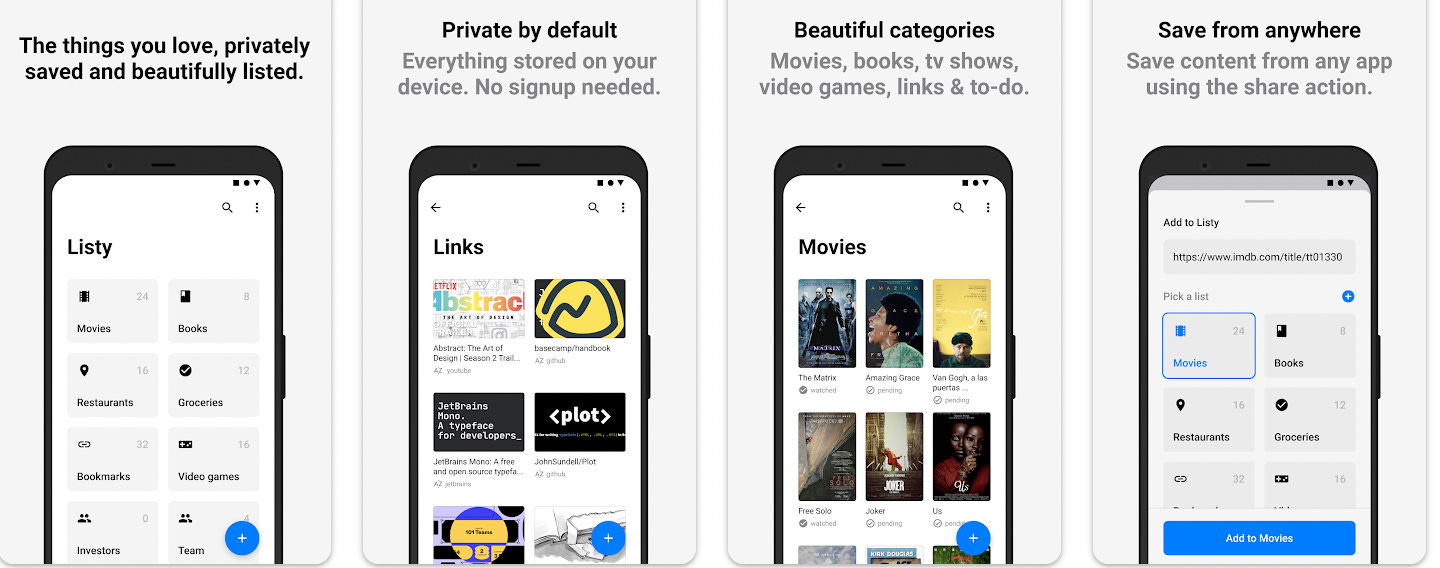The image is a collage of four horizontally aligned sections, each showcasing a cell phone screen with different app pages. From left to right, here is a detailed description of each section:

1. **First Section:**
   - **Header:** The top of the screen features black printed text stating, "The Things You Love, Privately Saved, and Beautifully Listed."
   - **Screen Content:** The phone displays a main page of an app called "Listie," which includes categories such as movies, books, restaurants, groceries, bookmarks, video games, investors, and teams. There is a blue circular button with a plus sign at the bottom.

2. **Second Section:**
   - **Header:** The black printed text at the top reads, "Private by Default."
   - **Subtext:** In gray text, it says, "Everything Stored on Your Device, No Sign Up Needed."
   - **Screen Content:** The phone shows a page with multiple picture boxes and hyperlinks, with another blue circular button featuring a plus sign at the bottom.

3. **Third Section:**
   - **Header:** The black printed text at the top reads, "Beautiful Categories."
   - **Subtext:** In gray text, it lists categories including "Movies, Books, TV Shows, Video Games, Links, and To Do."
   - **Screen Content:** The phone screen predominantly displays video thumbnails and, like the previous sections, a blue circular button with a plus sign at the bottom.

4. **Fourth Section:**
   - **Header:** At the top, the black text reads, "Save from Anywhere."
   - **Subtext:** In gray text, it explains, "Save Content from Any App Using the Share Action."
   - **Screen Content:** This section's phone screen illustrates features related to saving content across different applications.

Each section systematically highlights different functionalities and features of the "Listie" app, emphasizing privacy, category organization, and ease of saving content from various sources.